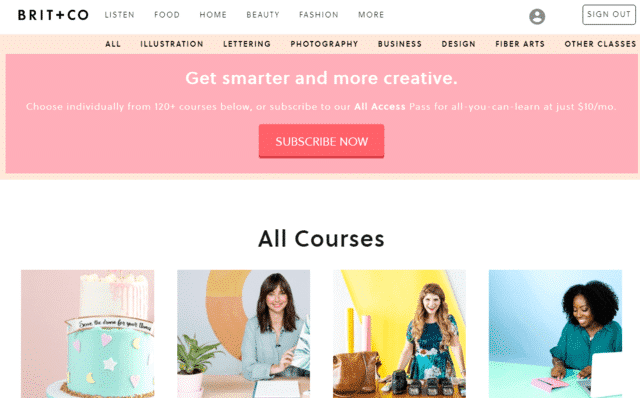The homepage of Brit + Co is attractively laid out to showcase the variety of online courses they offer. At the top, a sleek navigation bar includes links to sections such as Listen, Food, Home, Beauty, Fashion, and More. Directly beneath this is a submenu featuring specific categories like Illustration, Lettering, Photography, Business, Design, Fiber Arts, and other classes. The primary banner stands out with the inviting message, "Get smarter and more creative." It encourages visitors to "Choose individually from 120 courses below or subscribe to our All Access Pass for just $10 a month." This call-to-action is accentuated by a large, reddish-pink "Subscribe Now" button. 

Below the banner, the section labeled "All Courses" showcases four illustrative thumbnails: one featuring a cake, hinting at a bakery or cake decorating course; the second showing a woman with a houseplant, likely related to home decor; the third depicting a woman surrounded by cameras, pointing towards a photography course; and the fourth illustrating a woman with a notebook, suggesting a focus on writing, journalism, or general coursework. The design and content of the website aim to entice users to subscribe and explore Brit + Co's diverse range of creative courses.